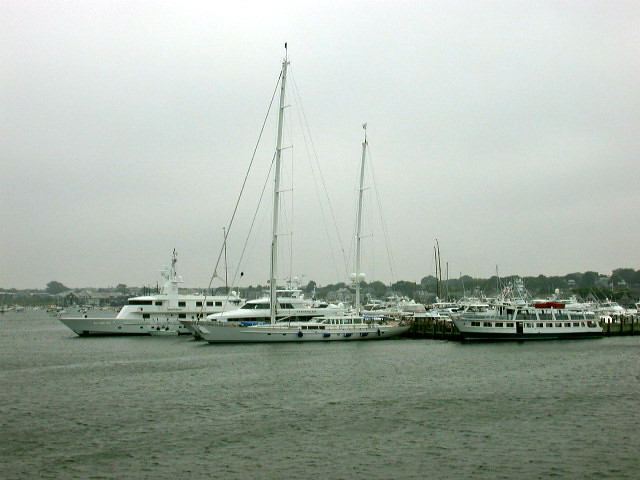The image captures a marina filled with a variety of large boats, including enormous sailboats and huge powerboats, all docked in the port on a gray, overcast day. The entire scene is tinged with a dull, cold, bluish hue, amplified by the gray sky and the rippling water, which shows a hint of wind. A house party boat is also docked, adding a unique touch to the array of stationary boats. The boats are predominantly white, with some having double decks and high rods for stability. In the distance, a mast wrapped in red stands out, and a white water tower with two containers is visible. The brown dock extends far out into the water, where some boats are moored. The horizon is lined with trees, contributing to the serene yet somber atmosphere. The overall image carries a slight blur, giving it an almost indistinct quality, while the predominant colors of white, blue, and gray blend seamlessly into the scene.